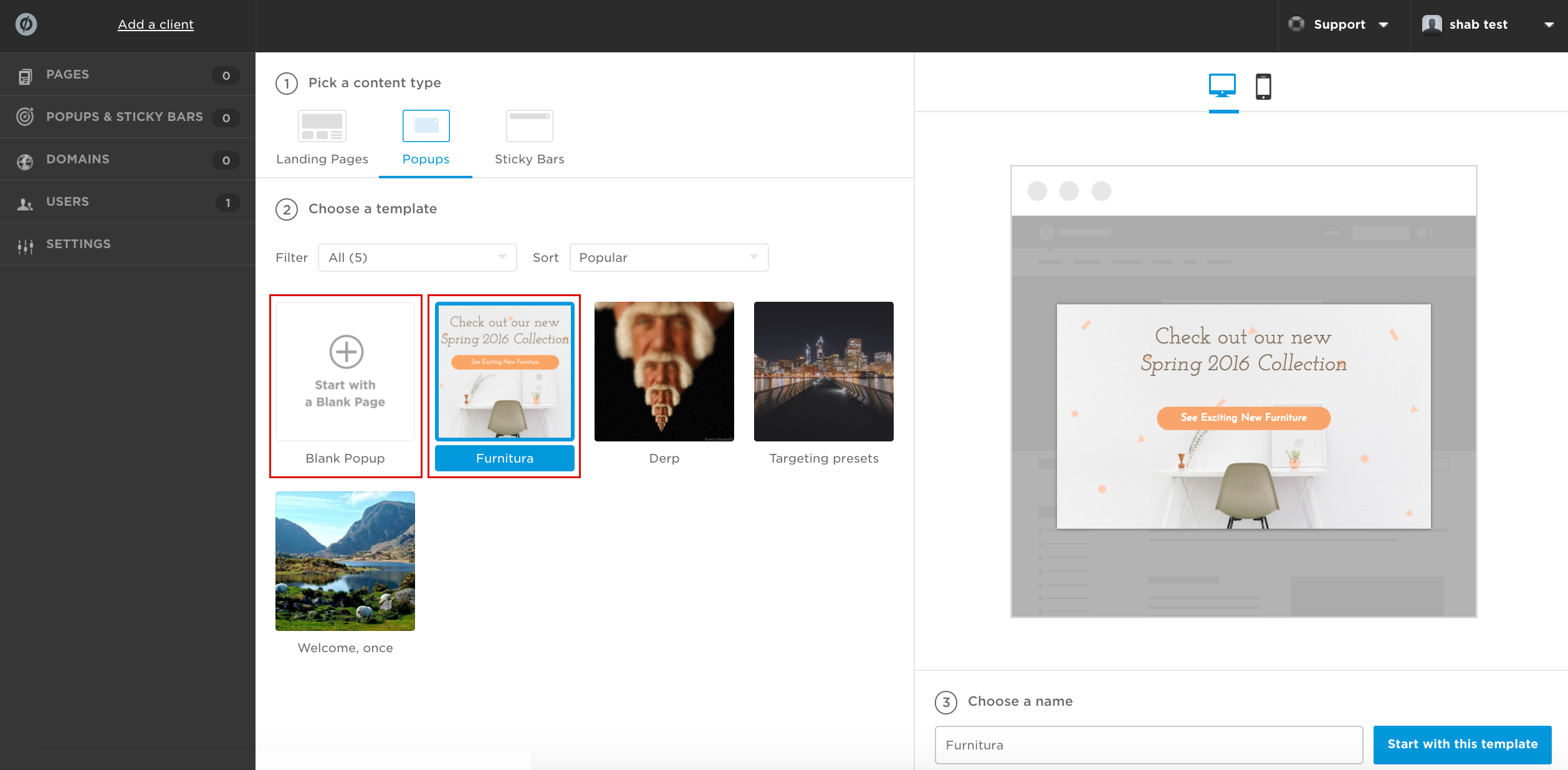In this detailed screenshot of a website application, the interface has a sleek design with black borders and dark gray accents. At the top, there's an underlined option reading "Add a Client," indicating it can be selected. Below this, there is an overview displaying various metrics: Pages (0), Pop-Ups & Sticky Bars (0), Domains (0), Users (1), and Settings.

The primary interface guides the user to first pick a content type from options such as Landing Pages, Pop-Ups, and Sticky Bars. In this instance, the user has opted for Pop-Ups. The next step involves choosing a template. The interface provides filtering options and the ability to sort templates by popularity.

One of the featured templates is titled "Furnitura" and includes an image promoting new furniture collections for spring 2016 with the caption, "Check out our new spring 2016 collections, the exciting new furniture." Additionally, another template image is humorously titled "Derp," featuring a meme of Hulk Hogan. The meme is notable for showing multiple descending images of Hulk Hogan with his iconic white beard appearing on top of his head, giving a whimsical touch.

Next to these templates, there is a section labeled "Targeting Presets," with a specific preset called "Welcome Once." The selected template "Furnitura" is shown zoomed in on the right side, demonstrating how it would look on both a webpage and a mobile phone. A support tab is visible, and the username displayed is "shab test." The user can input a name and begin with the selected template.